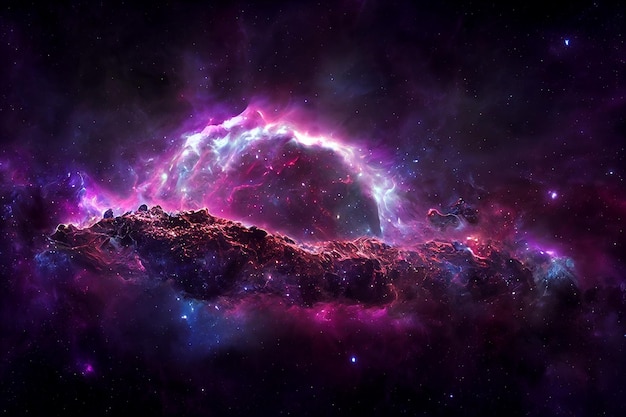This is a horizontally aligned rectangular image depicting a computer-generated scene of outer space. The four corners, as well as the top and bottom, are solid black, punctuated by scattered white and purple lights representing distant stars. Dominating the center is a large, rocky formation extending horizontally, with a rough, dark purple surface accented by hints of brown. Around this structure, wafts of almost ethereal purple smoke float gently.

Nestled within this formation, slightly to the upper middle part of the image, is a more rounded, planet-like rocky object. This celestial body showcases a striking blend of dark purple hues interspersed with vibrant pink highlights. Surrounding the object is a halo of white light swirls, lending it an illuminated, almost mystical aura. Above this planet-like structure, additional purple clouds emanate, dispersing across the black expanse and enhancing the otherworldly atmosphere.

The scene also features what appears to be a black hole or similar anomaly with purple and blue lights and occasional lightning-like bolts emanating from it, adding an even more dramatic element to the visual narrative. The entire composition is lit in such a way that parts of the objects seem to glow, creating a dynamic interplay between light and dark areas within the cosmic setting.